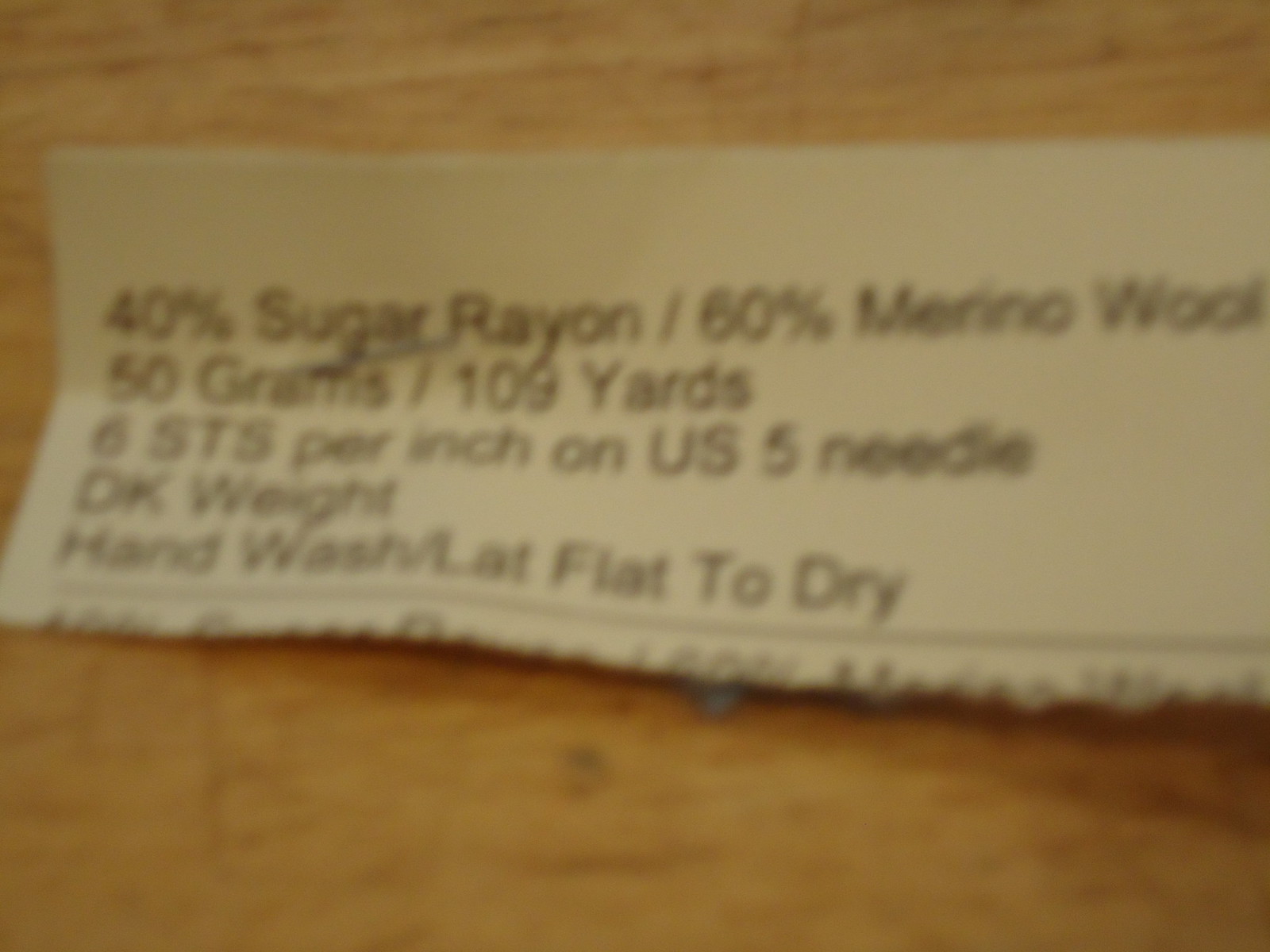The image depicts a somewhat blurry and possibly old digital picture taken indoors, showcasing a white rectangular label placed on a wooden dining table with a brown-black background. The label, with a texture indicative of specialist material, contains care and content information written in black text. The details on the label read: "40% sugar rayon / 60% merino wool, 50g / 109 yards, 6 sts per inch on US 5 needle, DK weight, hand wash / lay flat to dry." Notably, there is a small black line across the label, below which the text is partially obscured—possibly due to the paper being torn or folded.